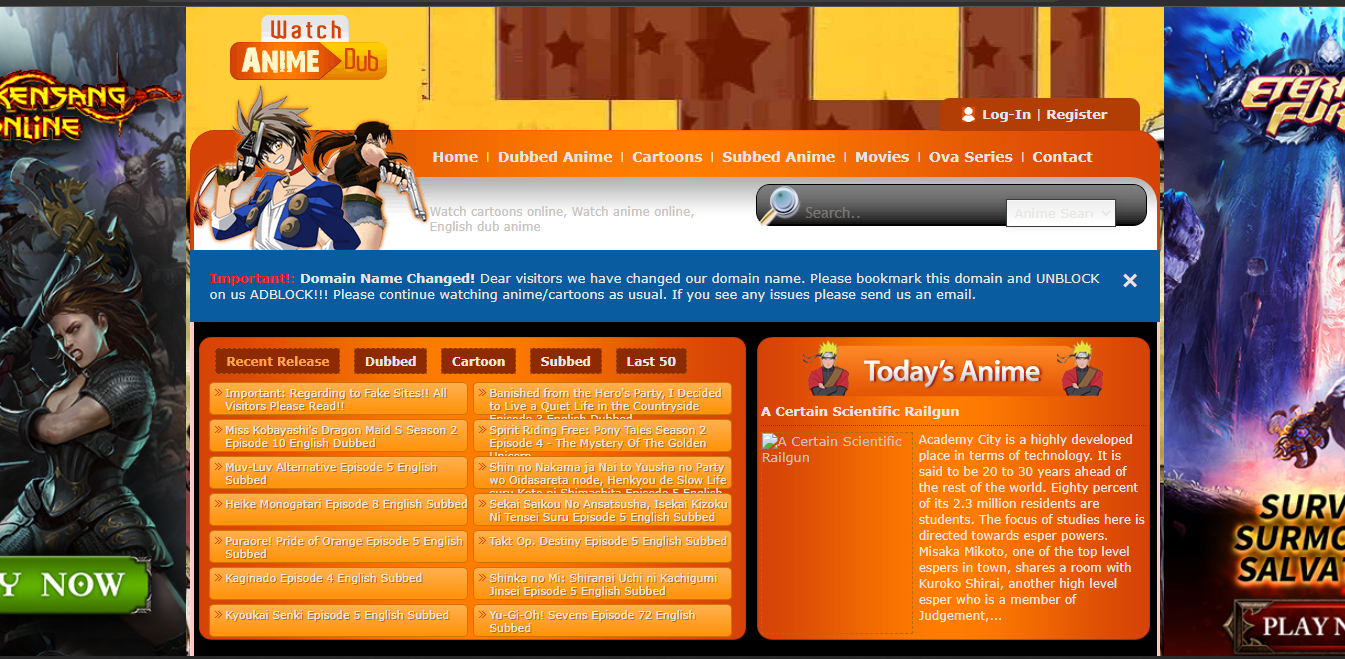#### Detailed Caption for a Vibrant Anime Website Image

Under the category of websites, this extremely colorful image features a vivid layout teeming with dynamic anime characters. The design includes two sidebars brimming with an array of anime figures. 

On the left sidebar, a warrior woman in intricately detailed armor, which notably has a low cut, is brandishing a double-headed axe amidst a backdrop that evokes fire and brimstone.

The right sidebar showcases a fantastical creature, rendered with a predominant palette of blue and pink hues, and possibly resembling a dinosaur. 

Centrally, the website bursts with bright yellow and orange tones. This section is populated by several anime characters, including a male figure with characteristic spiky hair and a vest, and a female figure in short shorts, both brandishing guns.

The text in the image reads a series of navigational and functional elements: "Watch Anime Dubbed," "Home," "Dubbed Anime," "Cartooned," "Subbed Anime," "Movies," "OVA Series," and "Contact." There are options to "Log In" or "Register," and a search function enabling users to find their favorite anime titles. 

Categories listed include "Recent Release," "Dubbed," "Cartooned," "Subbed," and the "Last 50." The highlighted anime of the day is "A Certain Scientific Railgun."